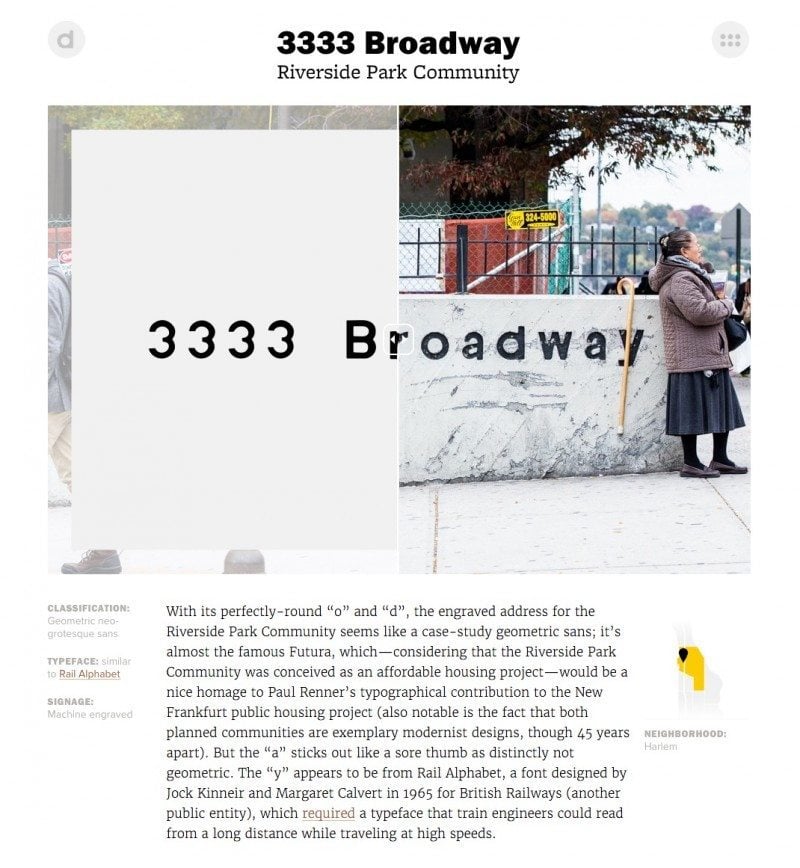This is an image of a website featuring the Riverside Park Community at 3333 Broadway. At the top left corner, there's a gray circle with a letter "D" inside it, while the upper right corner displays another gray circle containing six small gray dots arranged in a circular pattern. The focal point of the image is a photograph of a woman standing against a wall, seemingly in a park. The background reveals a tree enclosed by a red, white, and green fence.

The woman is dressed in a coat, a gray skirt, stockings, and shoes, with her hair styled in a ponytail. She is holding her pocketbook, and other people can be seen walking on the sidewalk behind her. Above the woman, the text "3333 Broadway" is prominently displayed across the picture.

Beneath the image, there's a detailed description discussing the geometric and architectural aspects of the Riverside Park Community. It highlights that the engraved address and the perfectly rounded O&D lettering draw inspiration from the geometric sands and the famous Futura typeface by Paul Renner. This typographical choice pays homage to Renner's contribution to the New Frankfurt Public Housing Project, noting that both planned communities represent exemplary modernist designs, despite being created 45 years apart.

On the right side of the webpage, there's an image featuring yellow and black elements, labeled with the term "classifications" on the left side of the section. The lower part of the description continues to elaborate on the new development in the Riverside Park Community area, indicating it may be a case study on affordable housing projects.